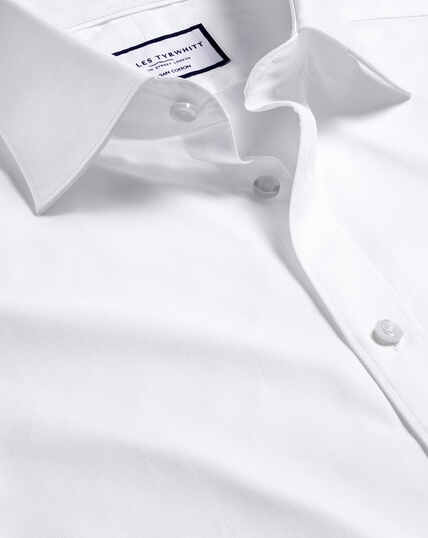This close-up photograph showcases a stark white button-down dress shirt, neatly laid flat with its collar spread to the sides. The shirt is slightly wrinkled, particularly around the chest area, despite appearing recently pressed, suggesting a high-end, yet realistic depiction of wear. The collar remains unbuttoned at both the throat and neck buttons, with only the third button from the top fastened. This detail highlights its readiness for pairing with a tie, typically suited for formal occasions. Centered on the back neck inside the collar, a label tag garners attention, featuring black bold text that appears to read “LESS TYRWHITT” within a black-bordered rectangle, though the smaller text remains illegible. The crispness and quality of the dress shirt hint at its high-end nature, aligning with the image's intimate focus on its craftsmanship.